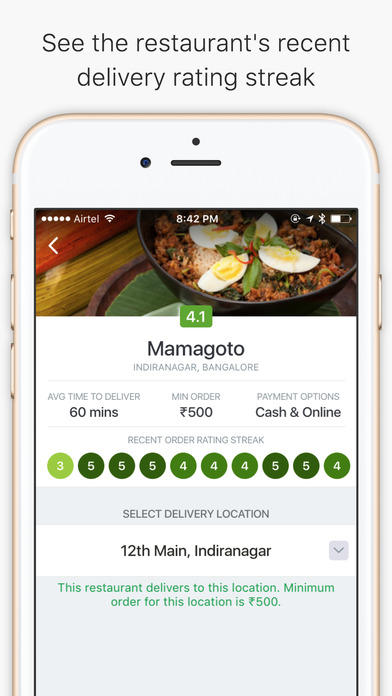This image is a screenshot of a food delivery app on a smartphone, presented in portrait orientation and shaped rectangularly, with dimensions approximately two to three times taller than it is wide. The background of the app is gray with a header in black font reading "See restaurant's recent delivery rating streak."

Central to the image is a depiction of a smartphone screen featuring an app interface. The phone's exterior has a pink border and a white top section. Displayed on the phone's screen is an enticing photograph of a dish, possibly a type of egg with meat underneath, served in a skillet.

At the top of the phone's screen are status indicators, including five signal dots, the label "Airtel," a full Wi-Fi signal meter, the time "8:42 PM," and icons representing Bluetooth, navigation, and battery status with a white meter.

Below the food image, a green box with white text displays the rating "4.1." The name "Mamagato" follows, with a location that appears to be "Indiranagar, Bangalore," although the name is not entirely clear. The text specifies an average delivery time of 60 minutes and a minimum order amount of 500, accompanied by an unfamiliar currency symbol. Payment methods listed are "Cash" and "Online."

Further down, the caption "Recent order rating streak" is displayed with a series of green text bubbles indicating ratings, which get darker as the numbers increase, ranging from three to five.